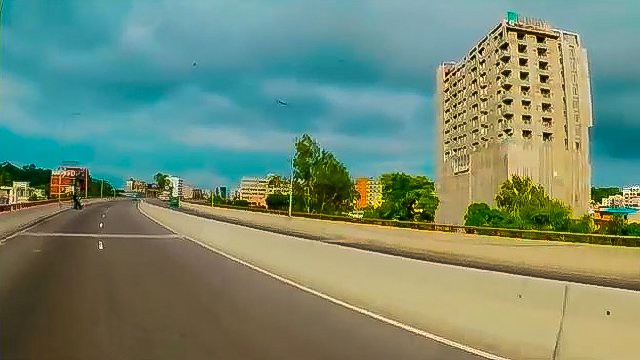A low-resolution, pixelated photograph captures an outdoor setting. The rectangular image, despite its poor quality, reveals a sky dominated by white clouds and patches of blue. In the bottom left corner, a dark gray road extends into the distance, bordered by white edges on both sides. Dominating the top right portion of the image is a tall, multi-level building with a tan facade.